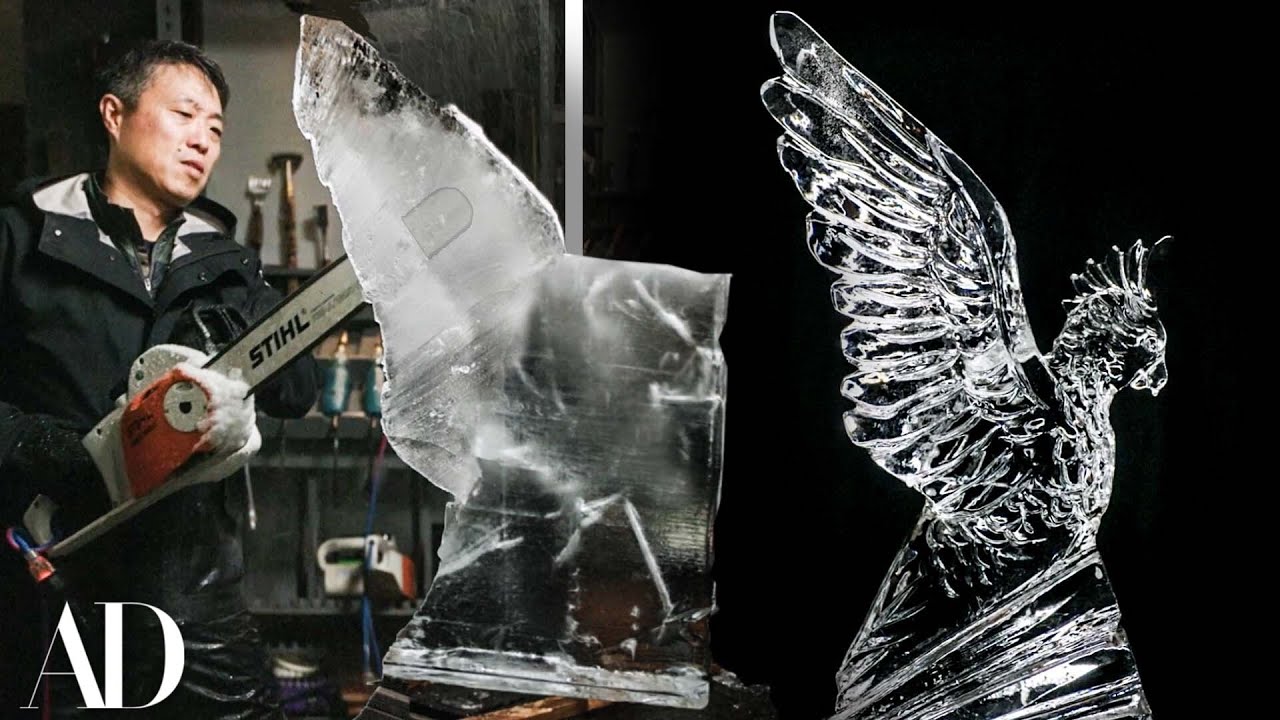In these photographs of ice sculptures, the left image captures an Asian man in a dark jacket using a STIHL chainsaw to meticulously carve a large block of ice. Prominently displayed at the bottom left are the bold white letters "AD." A silver-gray line divides the scene, with the left side highlighting the ongoing process of ice sculpting. The right side showcases the intricate completed sculpture of a bird with outstretched wings, decorated with five spherical adornments resembling a comb atop its head. The bird's detailed design and the contrasting black background emphasize its artistic elegance.